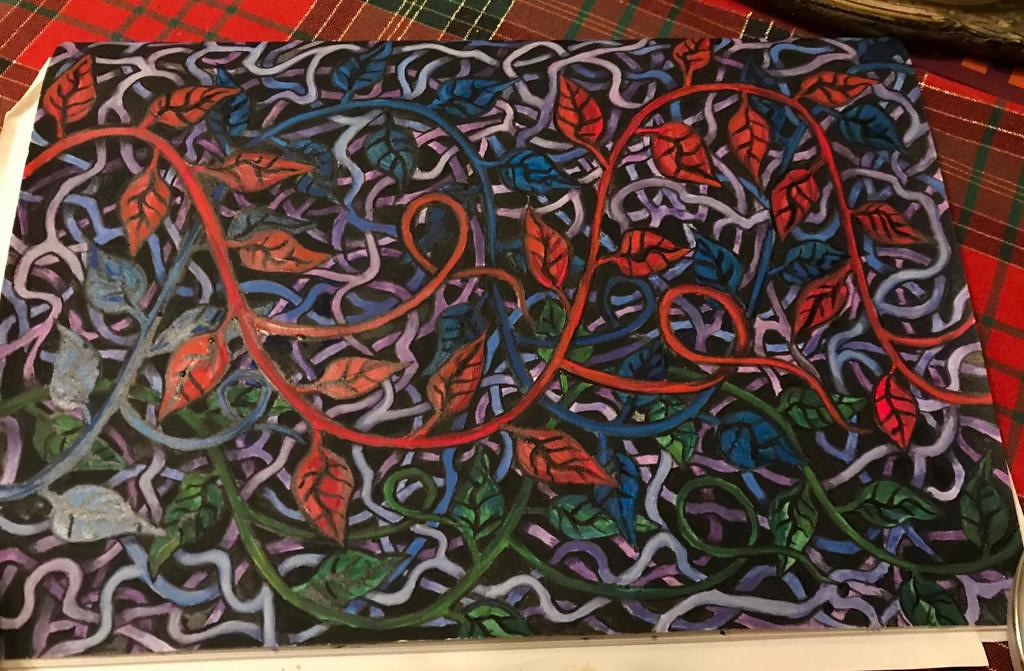The image showcases an intricate and highly complex work of art resting on a fabric surface. The fabric, possibly a tablecloth or comforter, features a plaid pattern in shades of red and maroon with thin silver stripes and wider black cross stripes.

The artwork itself is rendered on a sheet of paper, employing colored pencil and marker mediums. The sharpness and clarity of the edges preclude the use of crayon. The composition is a dense, interwoven array of vibrant colors, resembling tangled spaghetti. The intricate design includes red leaves with detailed veins, meandering along a winding red line reminiscent of a river. Hues of azure, light blue, green, and magenta further enrich the artwork.

Some leaves transition into a striking orange, blending seamlessly into a deeply tangled web of colored lines that span the entire piece, evoking the appearance of a complex chain-link fence. The background features a black surface that enhances the vivid colors overlaying it. The resulting effect is an extremely sophisticated and demanding masterpiece, reflecting sheer artistic brilliance.